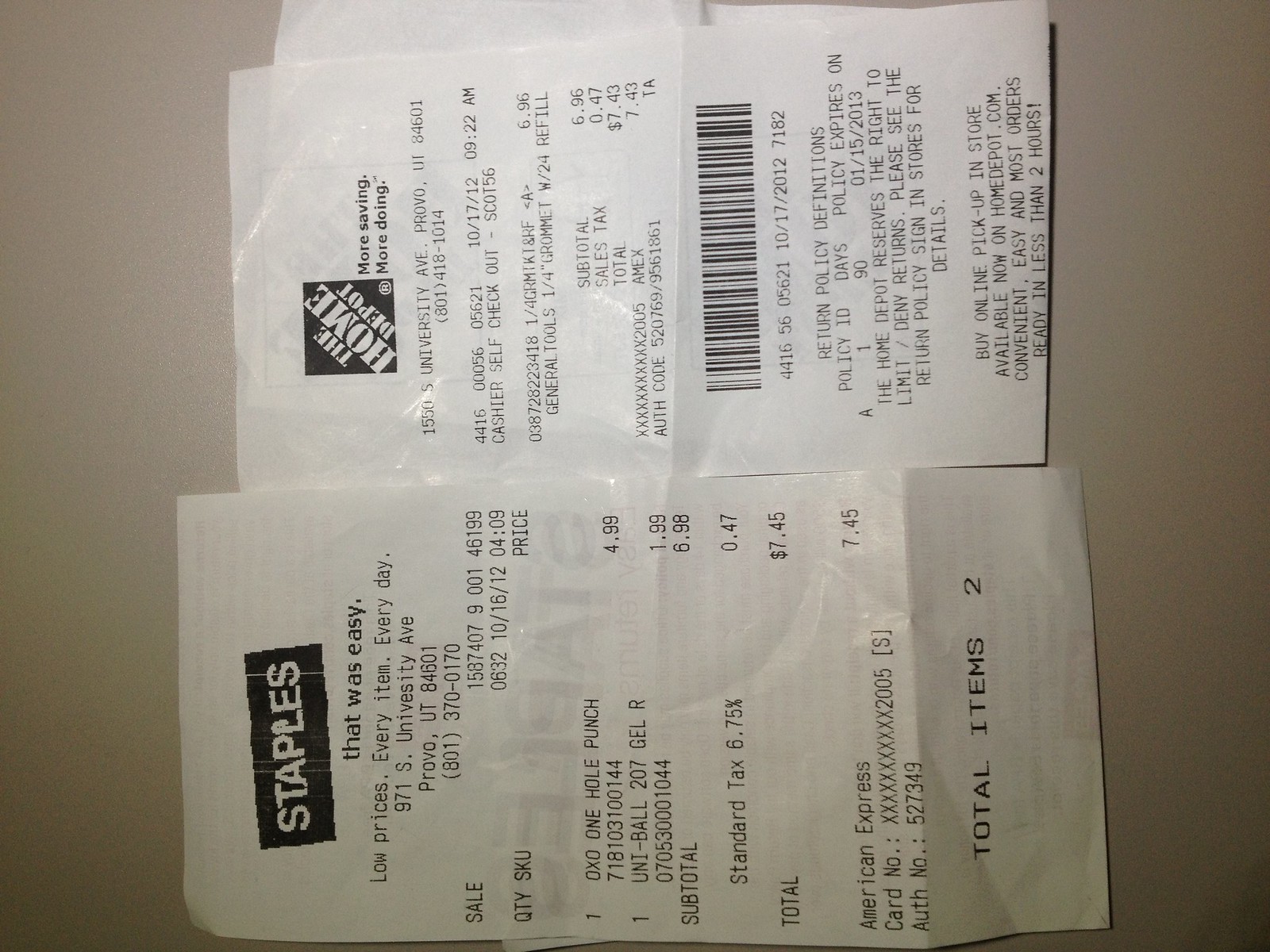The image depicts two black-and-white receipts laid out on a beige or brown surface, placed horizontally with their tops turned to the right. The receipts are slightly rotated, with the one from Staples located at the bottom and the one from Home Depot above it. Both receipts originate from Provo, Utah, and are dated from the year 2012. The Staples receipt shows a purchase total of $7.45 for a one-hole punch and a Uniball gel pen, and prominently displays the Staples logo alongside their taglines "that was easy" and "low prices every day." The Home Depot receipt, with a total of around $7.43, also features its logo and the tagline "more saving, more doing," indicating a purchase of some type of tool. Notably, both purchases were made using an Amex card.